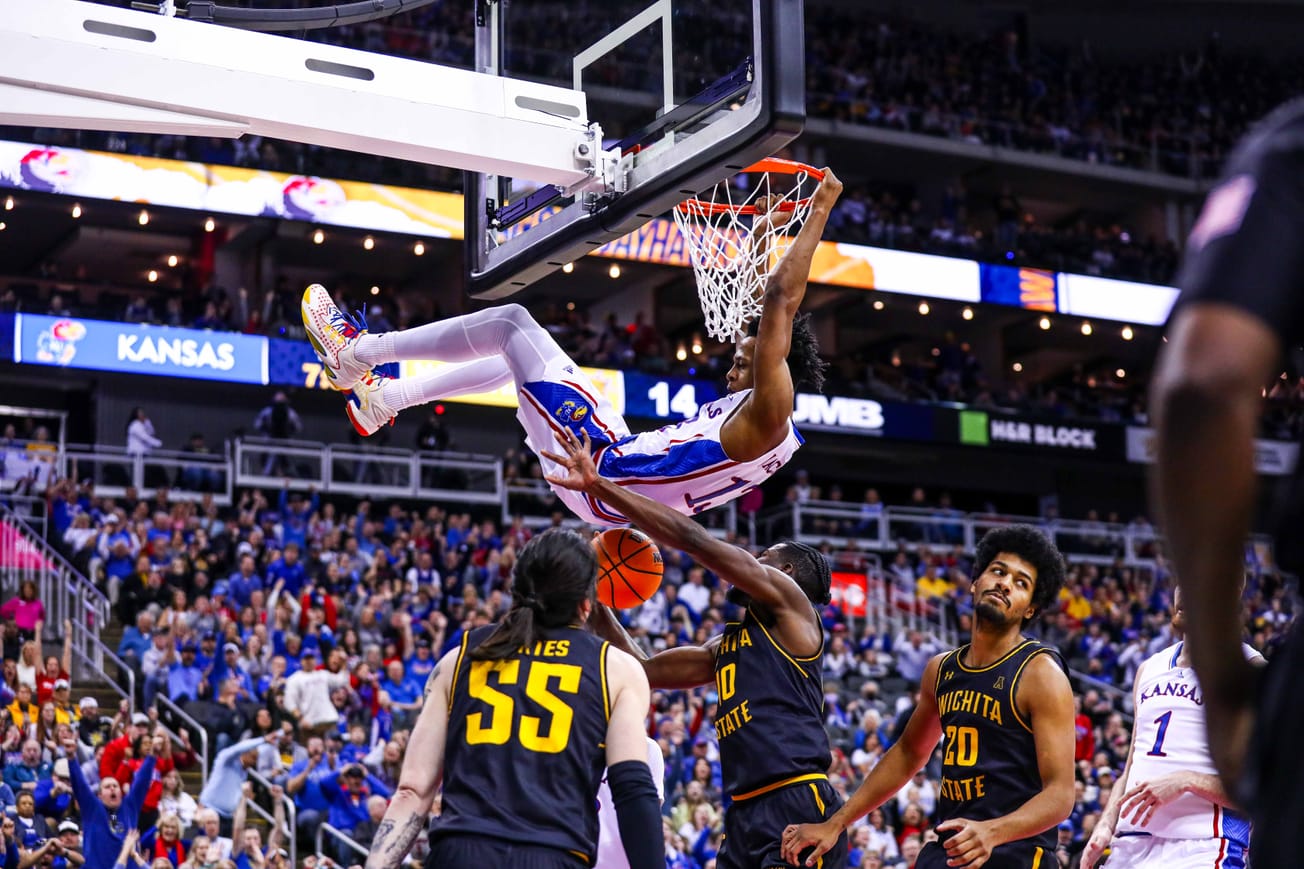In this vivid and dynamic color photograph taken from courtside during a thrilling basketball game, a Kansas player, donned in white and light blue, has just executed an electrifying slam dunk and is now hanging animatedly from the rim, his feet suspended in mid-air. Below him, three Wichita State players, clad in dark blue and yellow, are eagerly attempting to grab the ball. The packed stadium is bustling with energy, filled to the brim with fans, predominantly in blue, yellow, and white attire, suggesting a Kansas home game. The crowd in the background, a sea of colors, stands cheering in avid support, encapsulating the electric atmosphere of this live-action shot—a moment so vivid it could grace the front page of an old sports section or the cover of Sports Illustrated.